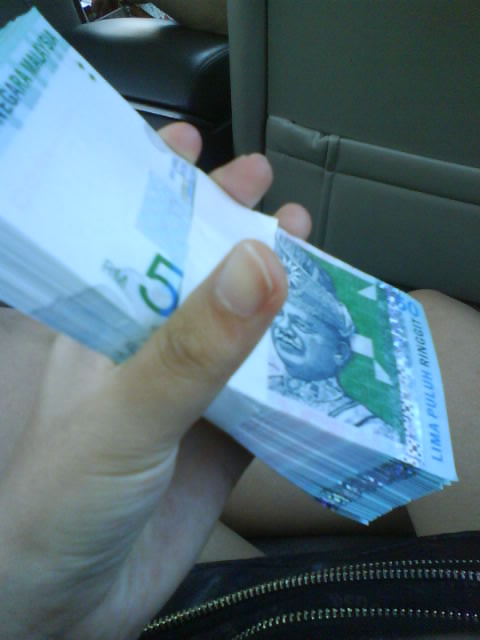In the image, a white adult female is seated inside a vehicle, perhaps an older car, as suggested by the visible center console and the leather seat with a pocket typically found on airline or car seats. She is holding a neatly wrapped stack of new foreign currency in her left hand, identifiable as Malaysian ringgit, with the label "Lima Pulum Ringgit" and featuring greens and blues in the design. Her thumb rests prominently on a white paper band around the stack, partially covering the number five. Beneath her hand, a black leather satchel, partially unzipped as if she had just retrieved the money, sits on her lap. Her clean, well-maintained fingernails indicate she likely does not work outdoors. The person's left leg is visible from the thigh to the mid-calf, pressed against the seat in front, adding to the close-up, detailed focus of the photograph.